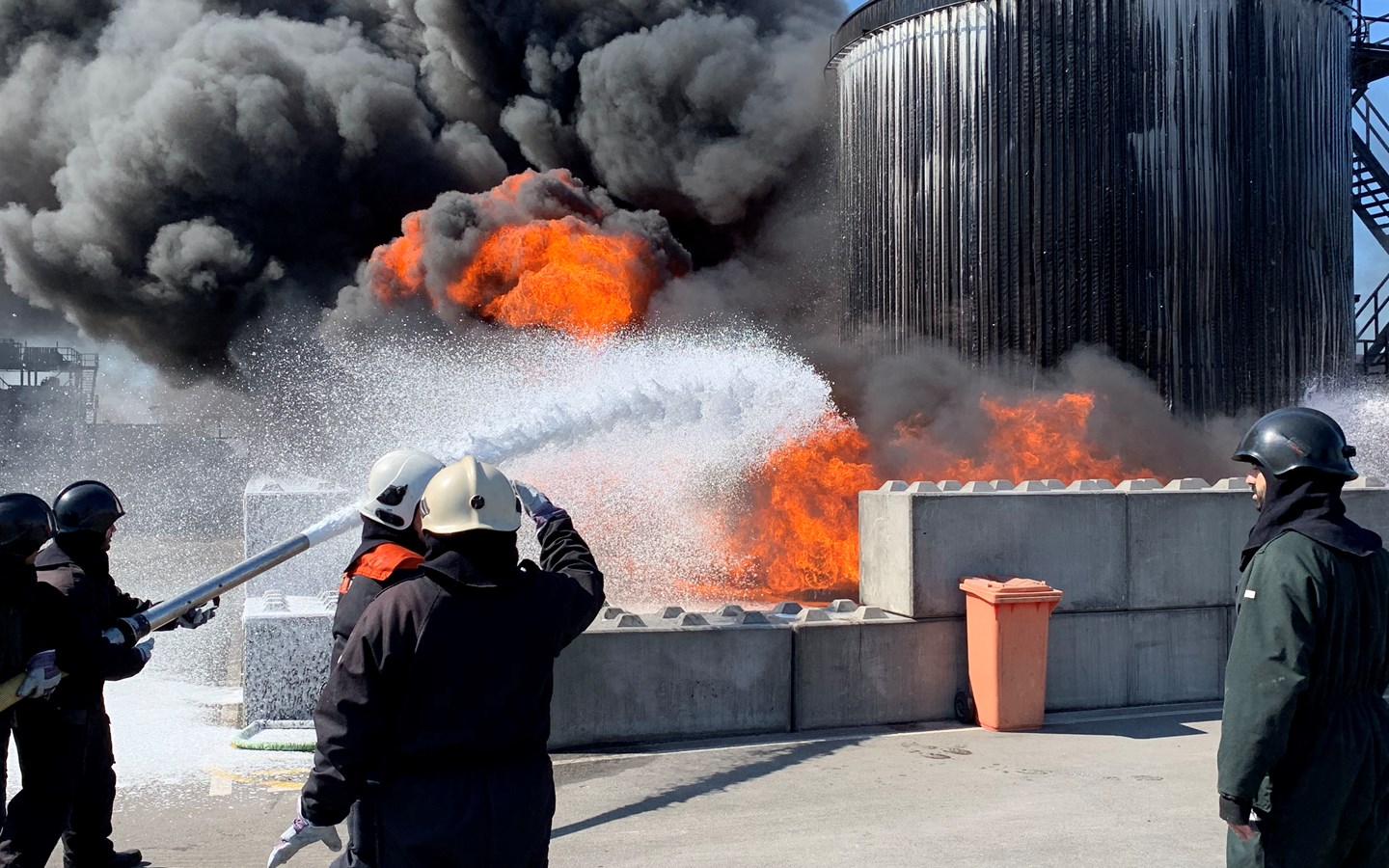In this dramatic scene, four firefighters, clad in helmets and long, fire-retardant coats, valiantly combat a raging fire engulfing a partly constructed or damaged building. On the left side of the image, a firefighter aims a hose emitting a foamy, white suppressant directly at the heart of the blaze. Two other firefighters stand nearby, observing the inferno intently; one in white gloves raises an arm towards the flames, perhaps signaling or directing efforts. The fourth firefighter stands to the bottom right of the frame, hands lowered, one casually touching his pocket, as he faces the destructive force. Orange flames and dark gray, billowing smoke dramatically contrast with the cinder blocks and the blackened structure behind them, highlighting the intensity and danger of the situation. The scene captures the dedication and bravery of these firefighters as they strive to control the disastrous blaze.